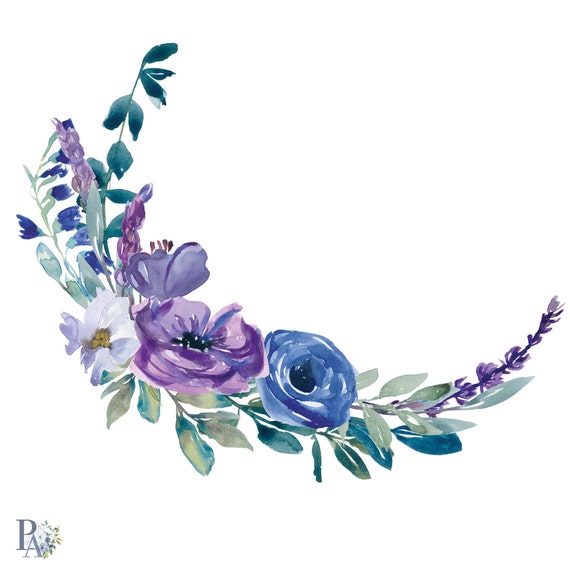This is an evocative watercolor painting that depicts a charming floral arrangement. The artwork prominently features an array of flowers and leaves, skillfully illustrated to form a crescent or U-shape with the open side pointing towards the top right. Positioned primarily in the bottom left, the composition includes an assortment of floral elements: a delicate white flower with a yellow center, vibrant purple flowers, a striking blue flower with a black center, and a cheerful yellow bloom. The leaves exhibit varying shades of green, from a light, fresh tone to a deep, forest green. Each element, though not overly detailed, contributes to the rich tapestry of colors, ranging from the blues and purples of the flowers to the greens of the foliage. Accompanying the floral display in the bottom left corner is the lettering "PA," which appears to be adorned with a small complementary floral motif, rendered in a similar watercolor style. The overall aesthetic evokes the gentle, handmade quality of a thank you card or a piece of refined stationery.